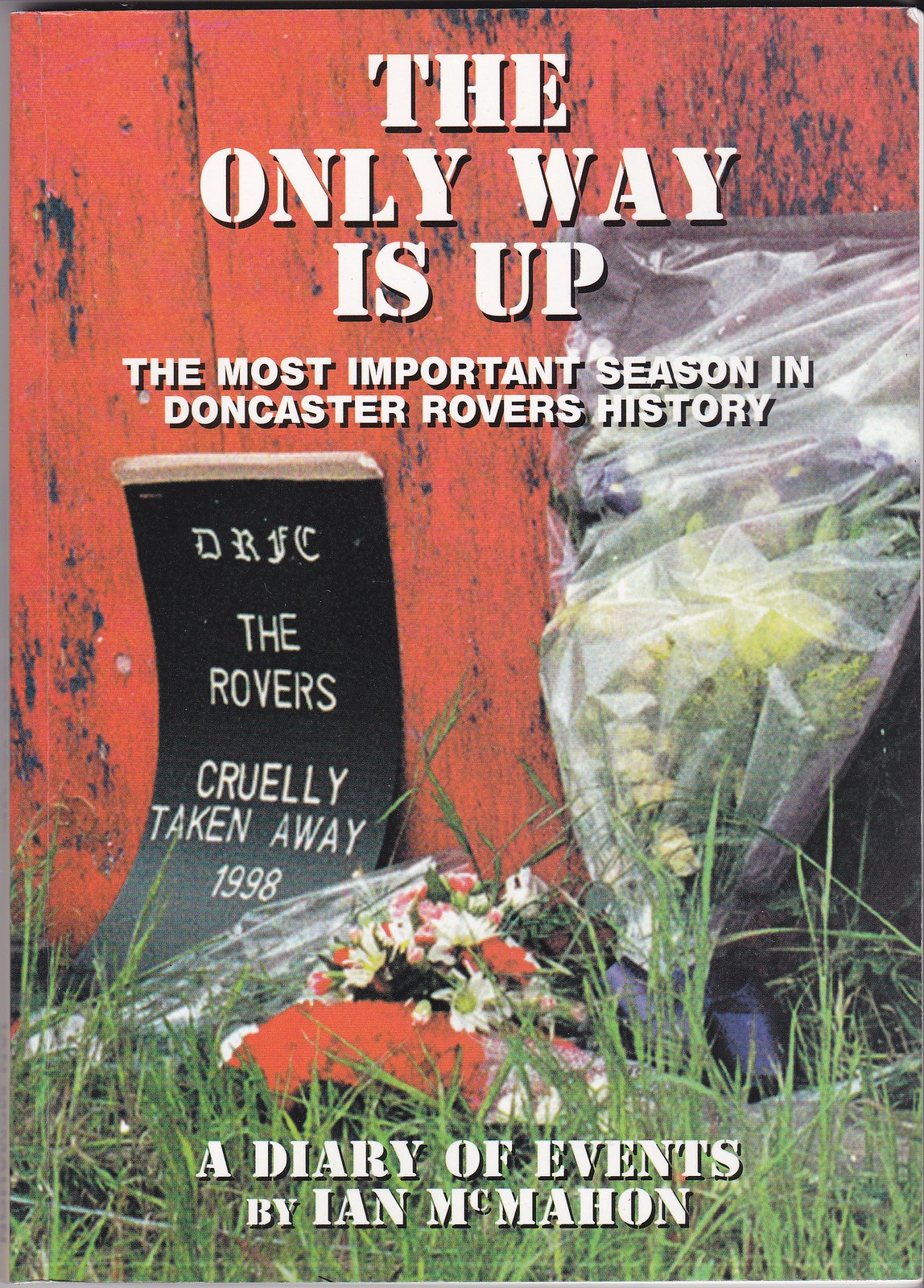The image depicts a book cover for "A Diary of Events by Ian McCann." Dominating the cover is the large, bold white title: "THE ONLY WAY IS UP: THE MOST IMPORTANT SEASON IN DONCASTER ROVERS HISTORY." Below this text is a somber scene featuring a black plaque that reads, "DRFC, the Rovers cruelly taken away in 1998." This plaque leans against a weathered red wooden wall, surrounded by bouquets of flowers placed in remembrance of a tragic event. The texture and color of the worn wall, along with the tall grass growing around the base, add to the poignant atmosphere of the cover.